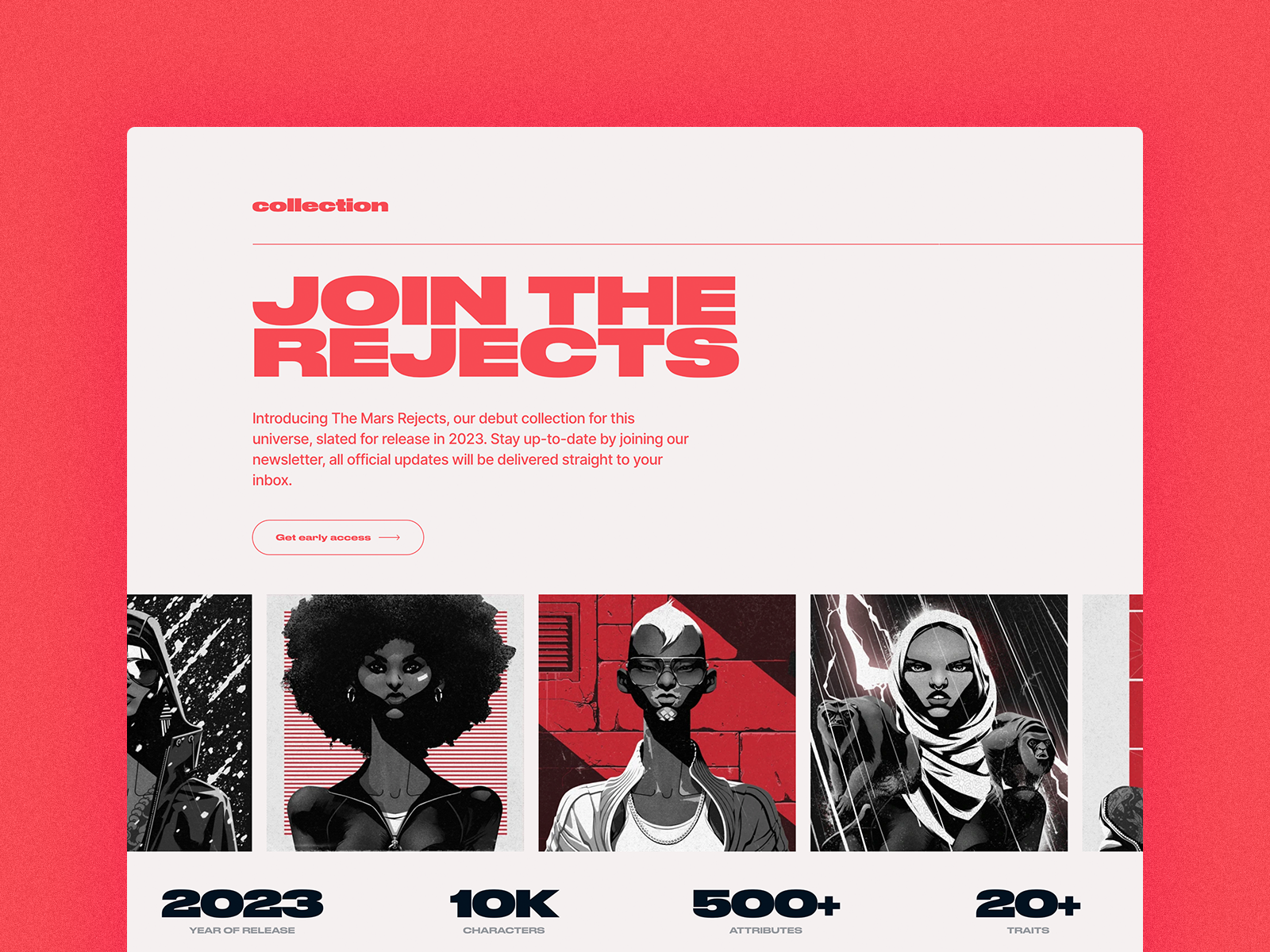The image features a design reminiscent of an album cover or an art collection promotion. It has a striking red border on three sides, resembling an upside-down U. This vivid red frame contrasts with a cream-tan background that occupies the interior space. In the top left corner, "Collection" is inscribed in the same shade of red, accompanied by a horizontal line that extends across the design. Dominating the center, bold and blocky red letters proclaim, "Join the Rejects: Introducing the Mars Rejects, our debut collection for this universe, slated for release in 2023. Stay up to date by joining our newsletter; all official updates will be delivered straight to your inbox."

Beneath this text are partially visible and full illustrations of cartoon or anime-style characters—three complete figures and a sliver of a fourth are discernible. Additionally, at the bottom, the image announces, "2023 year of release," alongside details like "10K characters," "500+ attributes," and "20+ [illegible text]." Although the exact nature of the collection is unclear, it hints at a possible video game or digital art project.